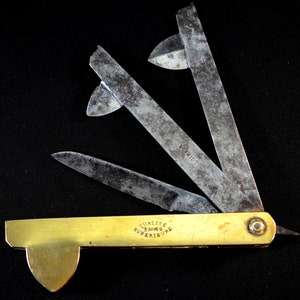This is a color photograph of an old Swiss Army knife, set against a solid black background. The handle of the knife is an aged gold color, featuring an unreadable printed text in the center, blurred and out of focus. Uniquely, the left side of the handle tapers into a pointed, spike-like extension. Emerging from the handle, which runs horizontally from left to right, are three oxidized metal tools, discolored with patches of black and silver, held together by a screw on the right side. The tools include a standard knife blade and two additional metal rods, each terminating in a shape reminiscent of an arrowhead or a single saw tooth, giving the impression of potentially being designed for puncturing or detailed cutting tasks. The overall scene is accentuated by the stark contrast between the black background and the gold, time-worn handle, highlighting the knife's vintage character.